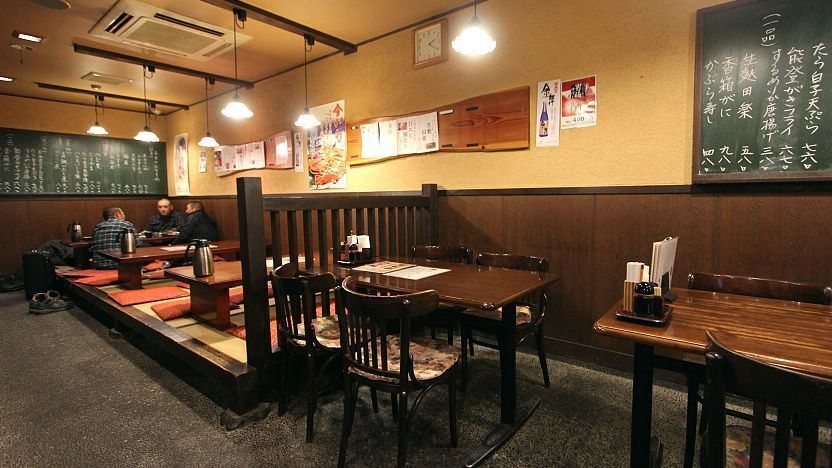The photograph captures the interior of a well-lit yet rustic Japanese restaurant. The space features two distinct seating arrangements: one with traditional low tables accompanied by cushions, where a group of three men are seated, possibly having a meeting or dining, and another section with standard wooden tables and chairs. The walls are adorned with vertical Japanese writing, including a green chalkboard with kanji above the men, contributing to the authentic ambiance. The decor is simple, with small lantern lights hanging from the ceiling, dark wood wainscoting, and various pictures or posters taped to the walls. The scene lacks visible restaurant staff or a visible kitchen, emphasizing an uncluttered dining environment. Each table is equipped with a menu, napkins, and likely condiments such as salt and pepper. The overall aesthetic is plain and somewhat dark, emphasizing functionality over elaborate decoration.